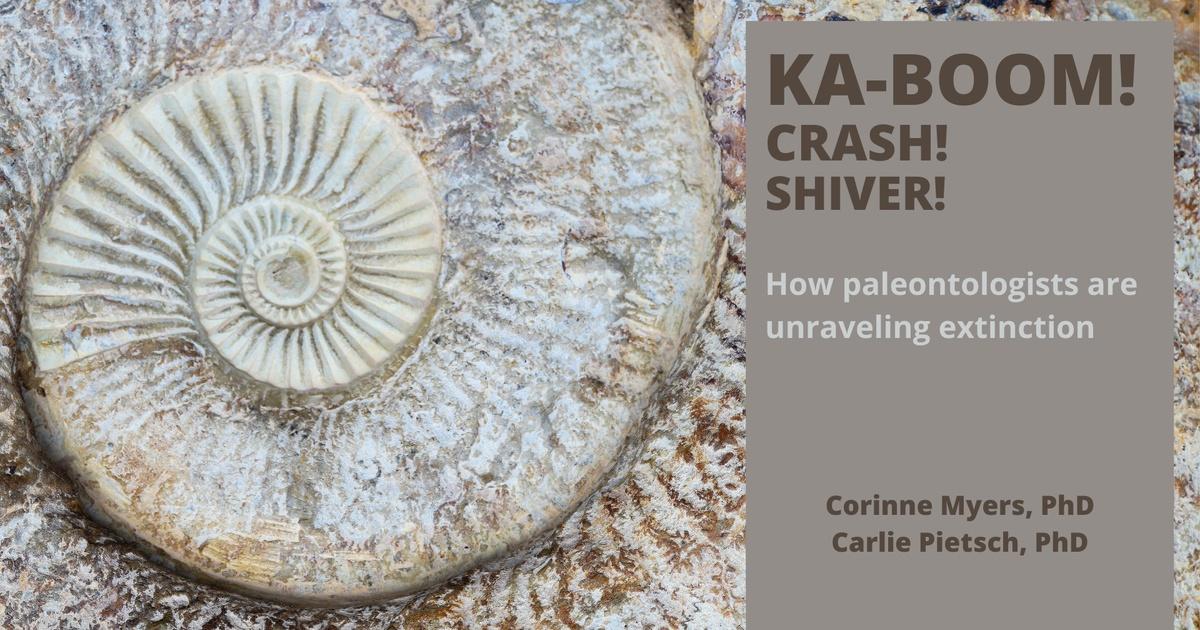The image depicts a PowerPoint slide related to paleontology. On the left side, there is a detailed photograph of a fossilized seashell that appears predominantly white with some gray and brown areas. The fossil showcases a spiraled, coiled structure, with intricate lines visible through its curves. On the right side of the slide, there is a gray rectangle containing black text that reads at the top, "Kaboom! Crash! Shiver!" followed by the subtitle, "How paleontologists are unraveling extinction." At the bottom of the text box, the names and titles "Corinne Myers, PhD" and "Carly Pietsch, PhD" are listed. The slide serves as an introduction to a scientific presentation on paleontology and the study of extinction events.